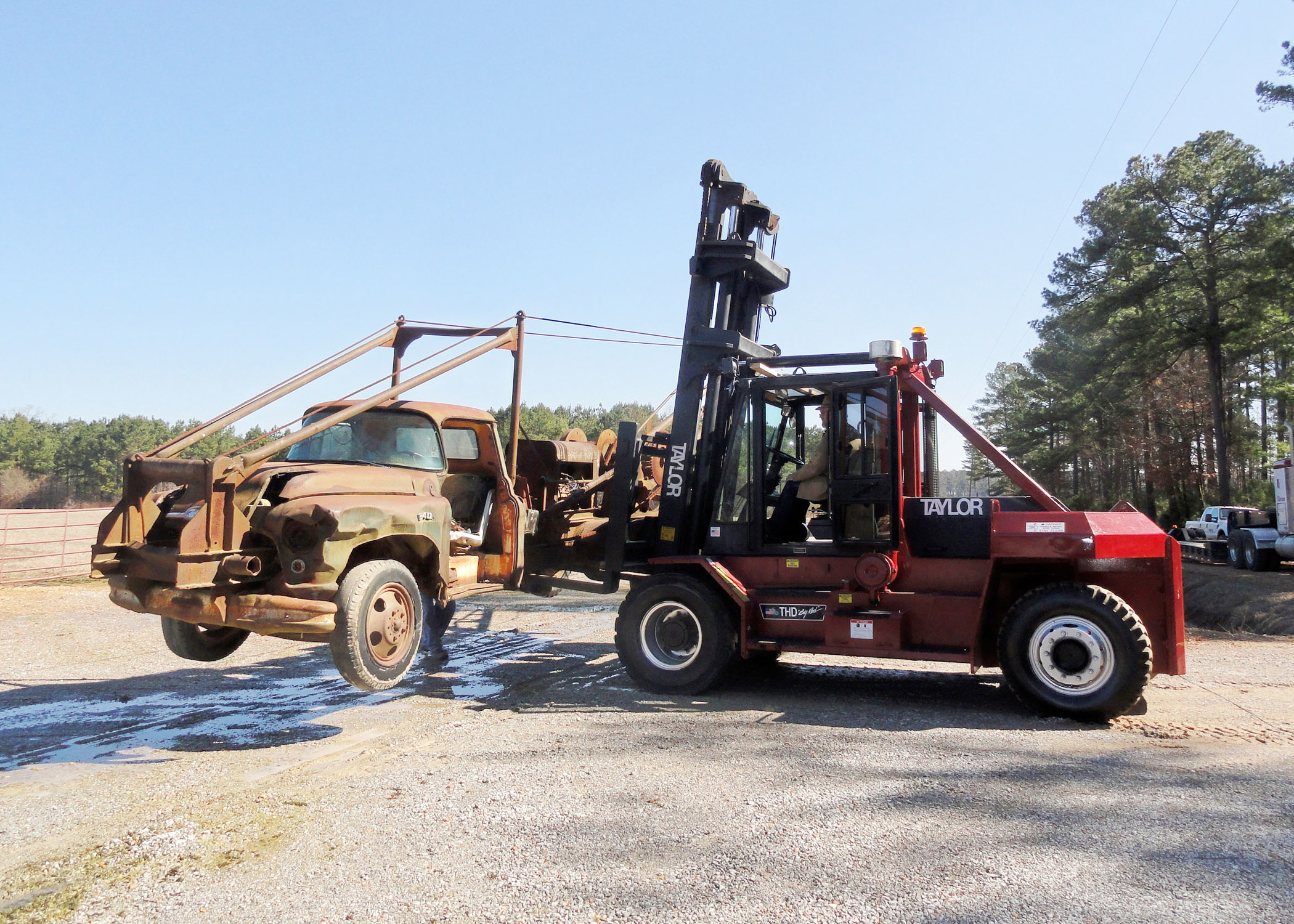In the image, a red Taylor-branded forklift, specifically designed for hefting heavy equipment, is in the process of elevating a significantly rusted, doorless vintage truck, likely from the 1940s or 1950s. The truck, reminiscent of models seen in the TV show "Sanford and Son," appears to be a well-worn work truck, possibly a tow truck, and is being secured with cables to prevent it from falling. The scene is set in an outdoor area with sandy pavement, surrounded by numerous pine trees and a clear, bright blue sky, indicating a sunny day following recent rain, as evidenced by the water and shadows on the ground. Additional vehicles can be seen in the background, possibly on a flatbed semi-truck, with one individual nearby overseeing the activity. The setting includes a gravel parking lot bordered by a fence on the left, emphasizing the industrious nature of the scene captured amidst a typical workday.